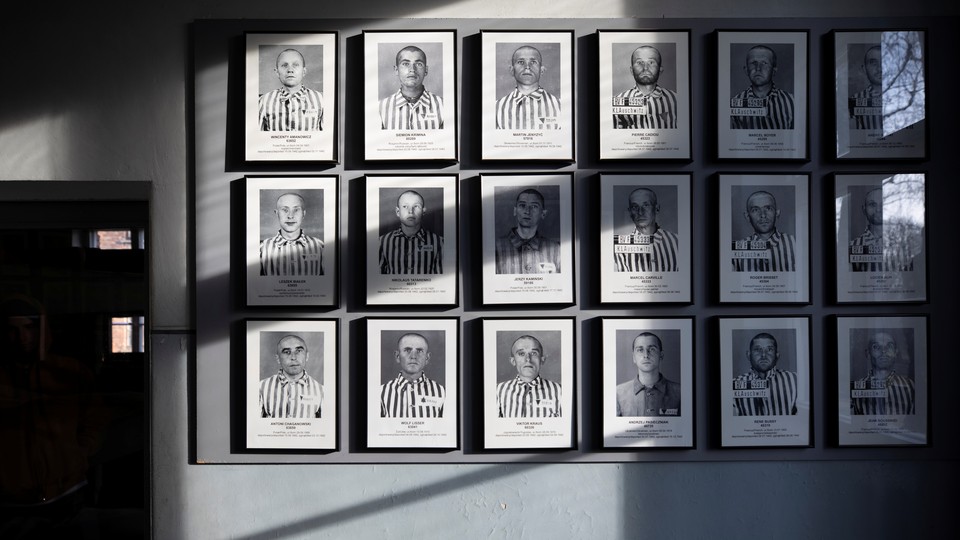The photograph captures a wall in a dimly lit room, showcasing 18 black-framed photographs arranged in six rows of three. Each frame contains a black and white image of men with shaved heads, wearing striped collared shirts reminiscent of prisoner uniforms from World War II. Small, barely legible names are inscribed under each photo, while a prison number is visibly placed next to each individual. The frames are mounted on a gray background that blends into the lighter gray, curved wall. The top right corner of the image reflects trees outside due to light streaming in through a nearby window. A shadow cuts through the center of the composition, and a doorway is visible to the left, enhancing the somber and reflective atmosphere of the scene.